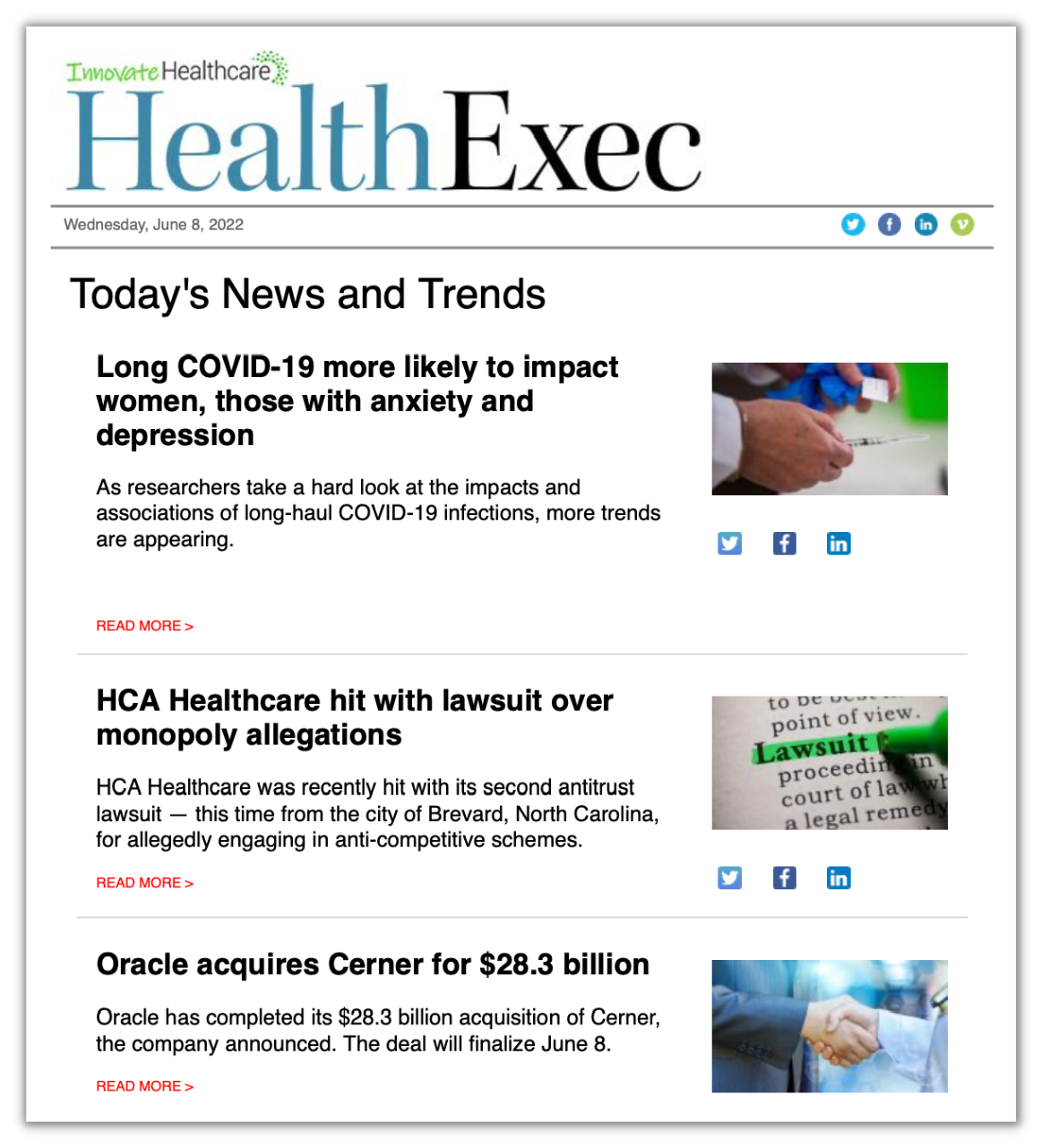"Health Exec Newsletter - Wednesday, June 8, 2022

At the top of this white-background newsletter, the title 'Health Exec' is prominently displayed, with 'Health' in blue and 'Exec' in black. In the upper left-hand corner, there is a logo in green and gray that reads 'Innovate Health Care'. Below the title, the date is clearly listed as Wednesday, June 8, 2022. To the right of the date, there are several social media icons arranged in circles, inviting readers to connect online.

Beneath the date, the newsletter is divided into three sections, each featuring an article overview with headlines followed by a small photograph to the right. The first article appears under the section titled 'Today's News and Trends'. The headline reads: 'Long COVID-19 More Likely to Impact Women, Those with Anxiety and Depression'. Next to this headline is a photograph depicting hands wearing long white sleeves holding a syringe, emphasizing the medical context. Beneath each article summary, there is some introductory text, with a 'Read More' link in red to encourage further reading.